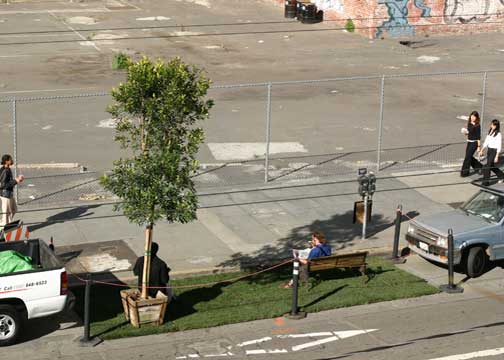The image captures a high-angle view of an urban scene featuring several distinct areas separated by clear boundaries. At the base of the composition, a street stretches from the lower left to the lower right, foregrounding the shot. Just above the street, a narrow patch of green grass hosts a small tree surrounded by a chain-link fence. To the left of this grassy area, a blue car with a faded hood is parked next to a parking meter. On the right, partially visible, are the tail end of a white truck and the front end of another car.

Beyond the grassy patch lies a wide sidewalk, bustling with activity. A woman in a blue jacket and tan pants sits on a bench near the center, possibly reading a newspaper. Two women walk side by side further to the right, and the middle of the sidewalk features a parking meter. The sidewalk itself appears somewhat unkempt.

In the background, behind the sidewalk and the chain-link fence, extends a large, cement-covered parking lot. Within this lot stands a pink building covered in graffiti, adding an element of urban grit to the overall scene. The photograph's arrangement provides a comprehensive view of this layered and lively urban environment.